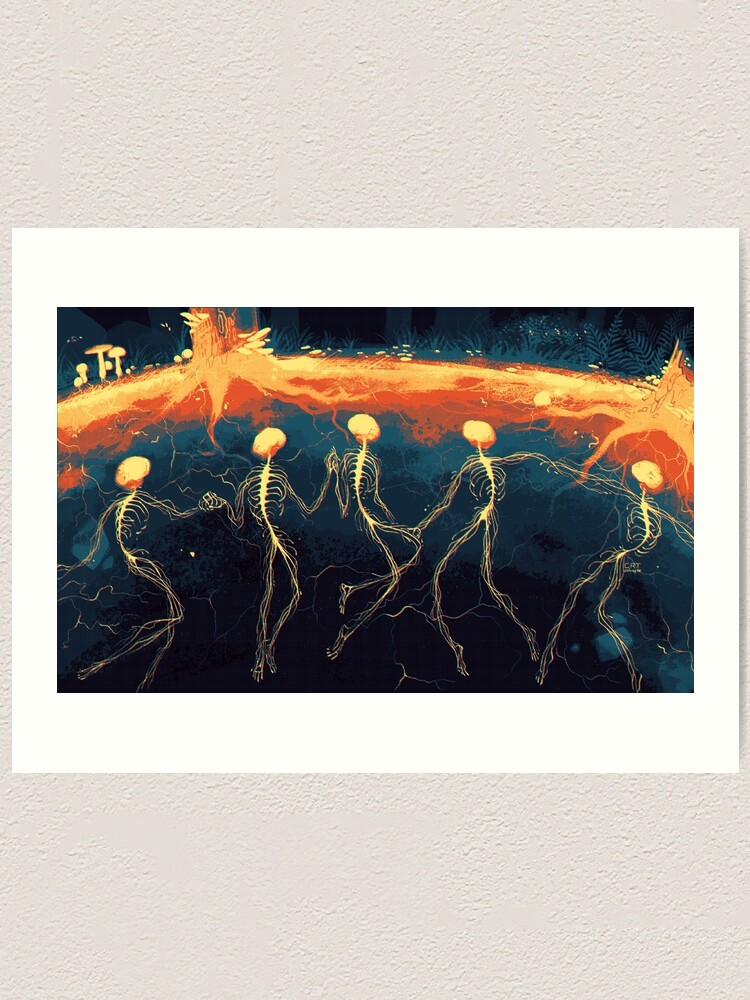The image is a surreal and impressionistic rectangular painting, set within a white frame and mounted on a cream-colored, textured wall. It depicts a dark blue background with shades that create a multi-layered effect. In the foreground, there are five very wispy, frail skeletons holding hands, appearing almost ethereal or spiritual with their long, wavy limbs and slender, wiry bodies. Each skeleton has a plain yellow head, which connects through their spinal columns, making them appear like spirits rather than typical skeletons.

Above the skeletons, an intense band of orange and yellow hues resembles a fiery supernova or molten lava cascading down, adding a sense of vibrant energy to the scene. In the top left corner, faint silhouettes of mushrooms and fern leaves are visible against the dark sky, giving the impression that the skeletons are underground or below the surface of the earth. The overall composition evokes a sense of otherworldliness, as if presenting a vision of spirits in the afterlife intertwined and dancing amidst a surreal, psychedelic landscape.